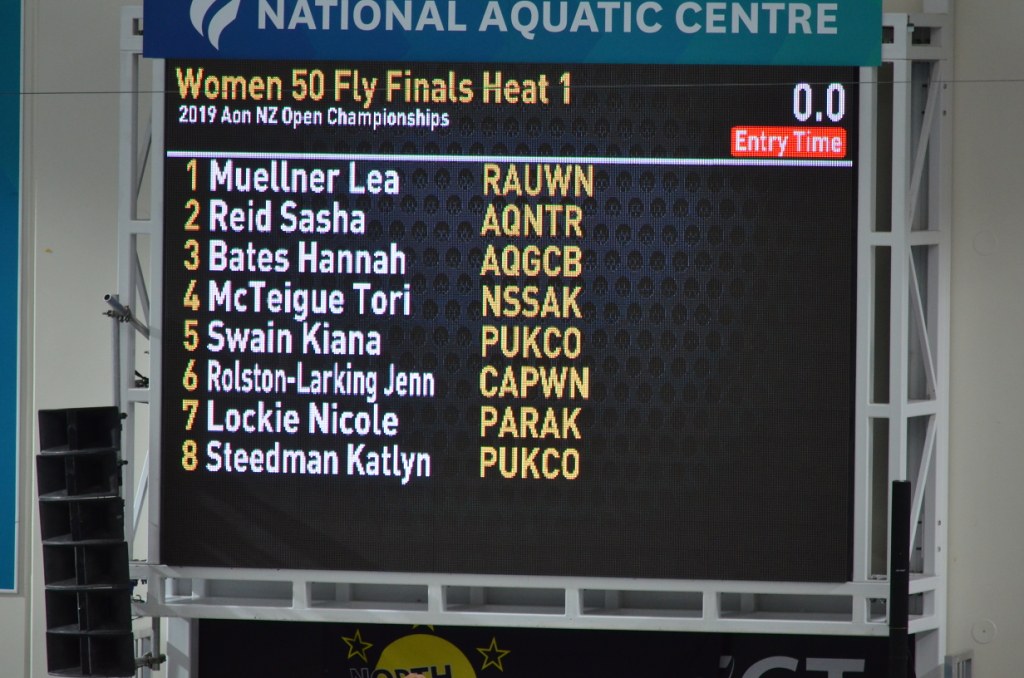This image displays a detailed scoreboard at the National Aquatic Center for the 2019 All-NCZ Open Championships. Centered in the scoreboard's blue header, "National Aquatic Center" is prominently written in white lettering. The event listed is the Women's 50 Fly Finals Heat 1. At the top right corner, the entry time is marked as 0.0, indicating that the race hasn't started yet. Below, there are eight competitors listed in white letters against a dark blue background, each swimmer paired with their respective team or identification letters in gold to the right. The participants are as follows: Miller Lear (RAUWN), Ray Shasha (AQNTR), Bass Hanner (AQGCB), Matigaudari (NSSAK), and Stephen Cayley (PUKCO). This scoreboard is brightly visible, ensuring all contestants and viewers at the event can see it clearly.